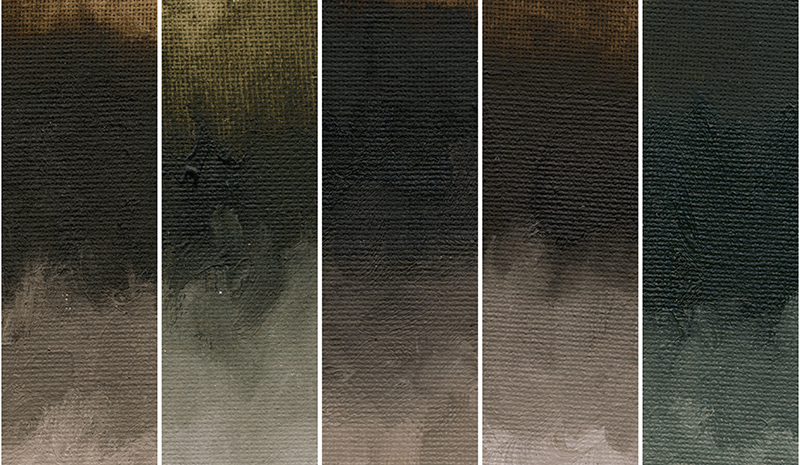The image depicts an abstract art piece comprised of five long, rectangular boards arranged side by side to form a single cohesive picture, suitable for displaying on a large wall behind a couch. The piece appears to be created with watercolor or possibly oil-based paint, and showcases a blend of colors including dark gray, blue, white, tan, cream, and pinkish hues. The boards vary in their gradient, with most transitioning from lighter tones at the bottom to darker shades at the top. The first, third, fourth, and fifth boards are notably darker, with the fifth board being the darkest. Some boards reveal the light brown or tan canvas partially. Intricate details include smoky gray at the bottom of several panels and sections where the darker hues concentrate at the top, creating a dramatic and moody effect. The art features no accompanying text and is distinguished by a series of brush strokes and color gradients, manifesting the artist's vision in a divided yet unified format.